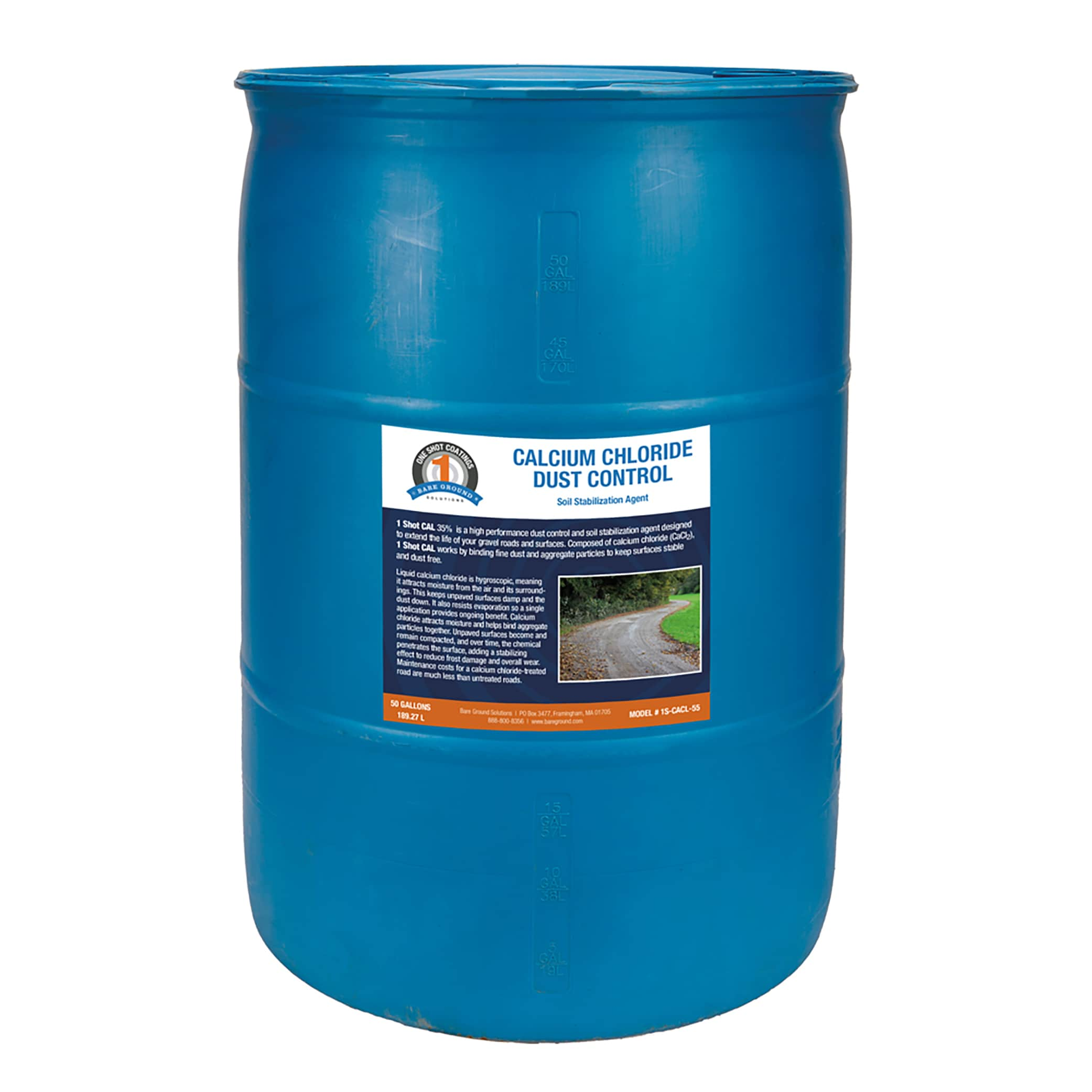The image shows a large, light blue, cylindrical 50-gallon plastic drum with a round top and distinct ridges one-third and two-thirds of the way down. The drum has a label in the middle, prominently featuring a white section at the top with blue text that reads "Calcium Chloride Dust Control Soil Stabilization Agent." To the left of this text is an emblem consisting of half a black circle with an orange number one inside it, and a blue band underneath that is too small to read. Below the white section, there is a dark blue area with two paragraphs of text that are also too small to decipher, likely containing usage instructions or product information. Positioned to the right of this text is a picture of a dirt road flanked by trees on one side and grass on the other. At the bottom of the label is an orange bar with white text, which is similarly unreadable. The overall color of the drum is described as a true, ocean-like blue, and it resembles a container that might be used for storing rainwater or seen in crime shows.